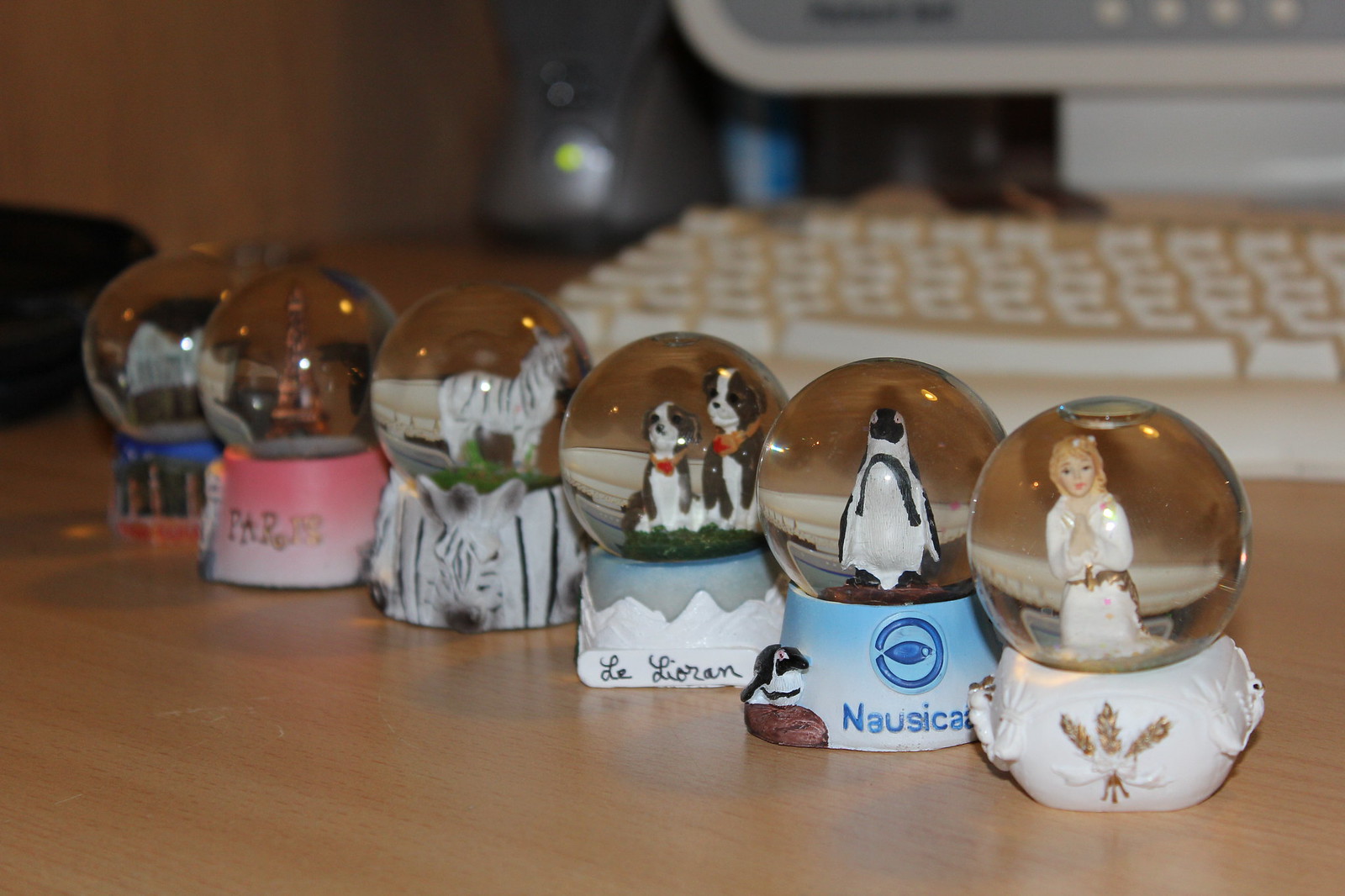The image is a color photograph taken indoors under artificial lighting, showcasing a fascinating collection of six snow globes arranged in a line on a blonde wood table, receding into the background. The snow globes move from the right bottom portion of the image to the center left, starting with the one closest to the viewer, which is sharply in focus, gradually becoming less focused towards the back. 

The foremost snow globe features a white ceramic base adorned with gold flowers and wheat stalks tied with a ribbon, encasing a figure of an angelic woman with blonde hair, clad in a white dress or robe with a gold sash. The second globe has a blue base fading to white, decorated with a logo of a circle and fish, bearing the name "Nausicaa." Inside, it contains a penguin figure. Following this is a snow globe with a gray and white base resembling snow-covered mountains, with the name "Leoran" inscribed on it, containing two spaniel dogs with red collars.

The fourth globe features a zebra, both in the globe and on its base, which is intricately designed to mirror zebra stripes. The fifth globe has a pink base with a depiction of the Eiffel Tower inside, hinting at its Parisian origin. The final snow globe, though less distinct, has a base with blue at the top, red at the bottom, and possibly black and gold stripes in between, with unrecognizable portions inside the globe itself.

In the blurred background, there is a cream-colored keyboard, the top portion of a computer monitor, and the bottom part of a gray desktop computer, adding a subtle technological contrast to the nostalgic snow globes in the foreground.